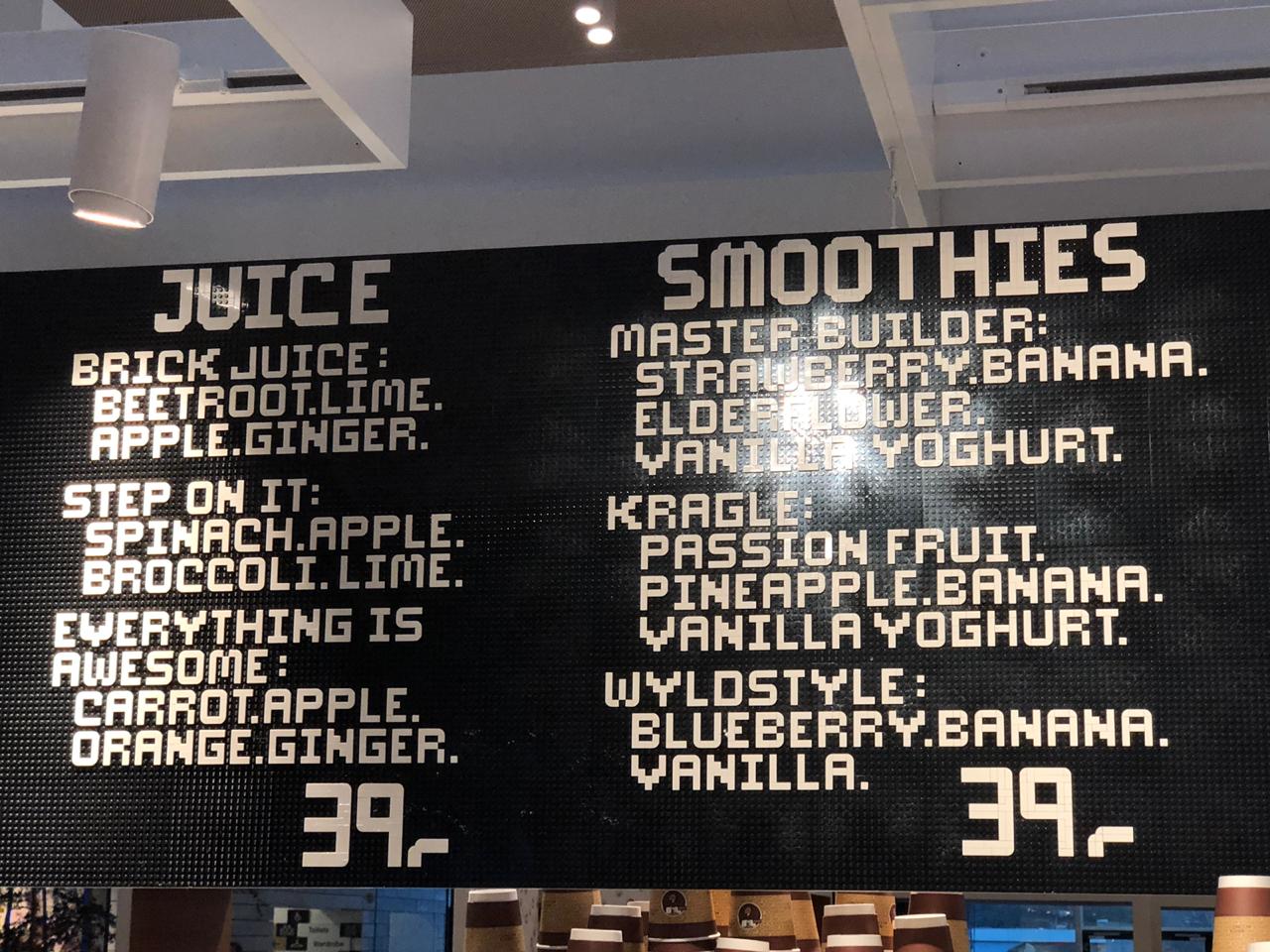The image is predominantly occupied by a large, black menu board, centrally placed in what appears to be a juice bar. The board, displaying white text, is illuminated by lights installed within square or rectangular frameworks in the white-blue ceiling above. The left column, titled "Juice" in bold font, lists three juice combinations: "Brick Juice" (beetroot, lime, apple, ginger), "Step on It" (spinach, apple, broccoli, lime), and "Everything is Awesome" (carrot, apple, orange, ginger), each priced at $39. On the right, the "Smoothies" column showcases "Master Builder" (strawberry, banana, elderflower, vanilla yogurt), "Kregel" (passion fruit, pineapple, banana, vanilla yogurt), and "Wild Style" (blueberry, banana, vanilla), also priced at $39. The menu surface has a mesh-like texture, with a sun reflection partially obscuring some text. Below the board, a sliver of the room is visible, showing a few stacked brown paper cups and indistinct background elements.